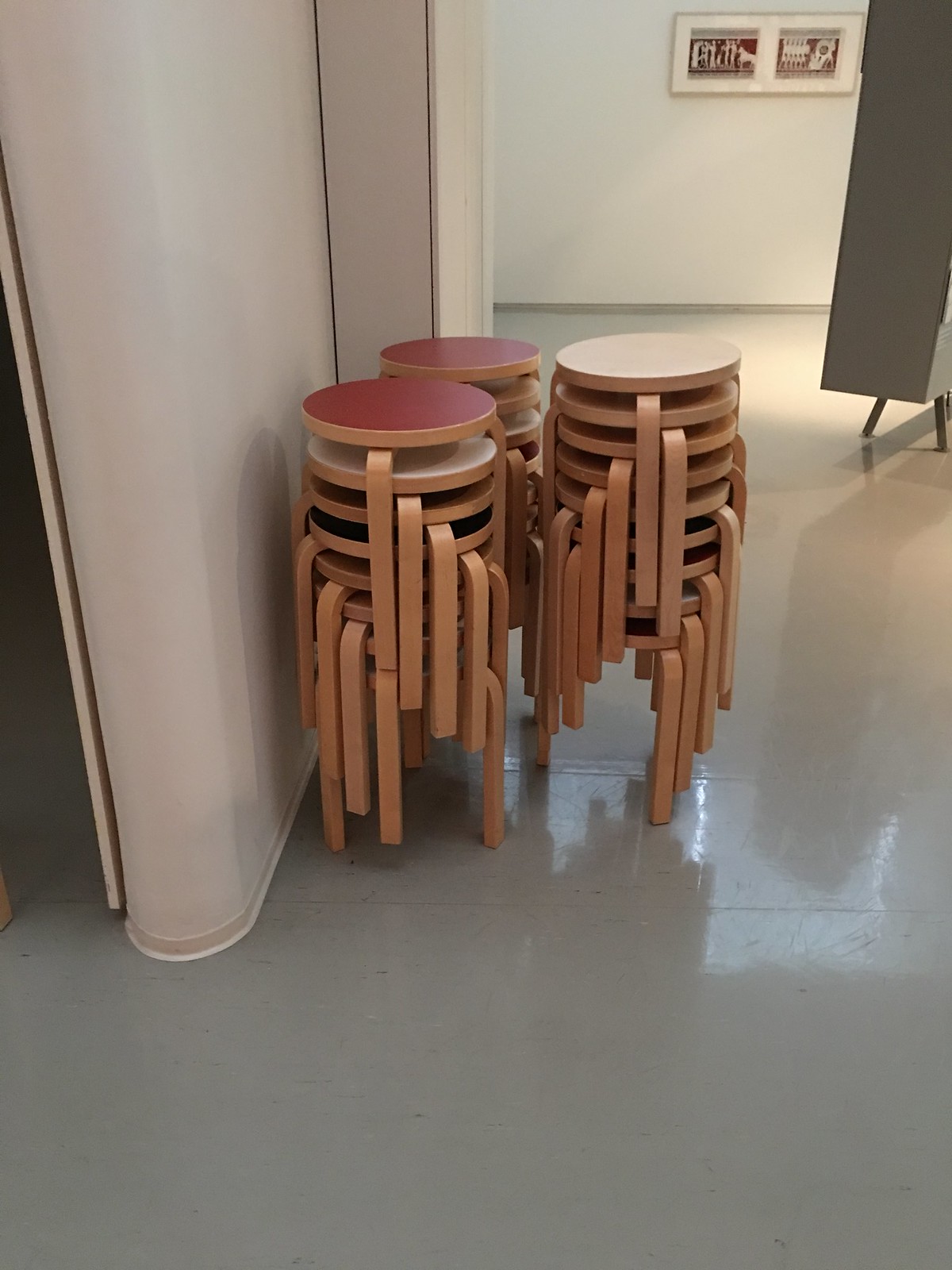This is a color photograph of an indoor setting showcasing three stacks of round, wooden stools with flat tops. The stools are primarily light wood in color, with some having burgundy tops and one having a white top. Positioned diagonally, they stand prominently in the center of the image. The backdrop consists of a beige and blue wall to the left and a shiny, white, reflective floor below. A piece of framed art is visible in the top right corner, although the details of the artwork are unclear. The overall composition of the photograph is rectangular, focusing mainly on the stacks of stools against a simple, understated background.